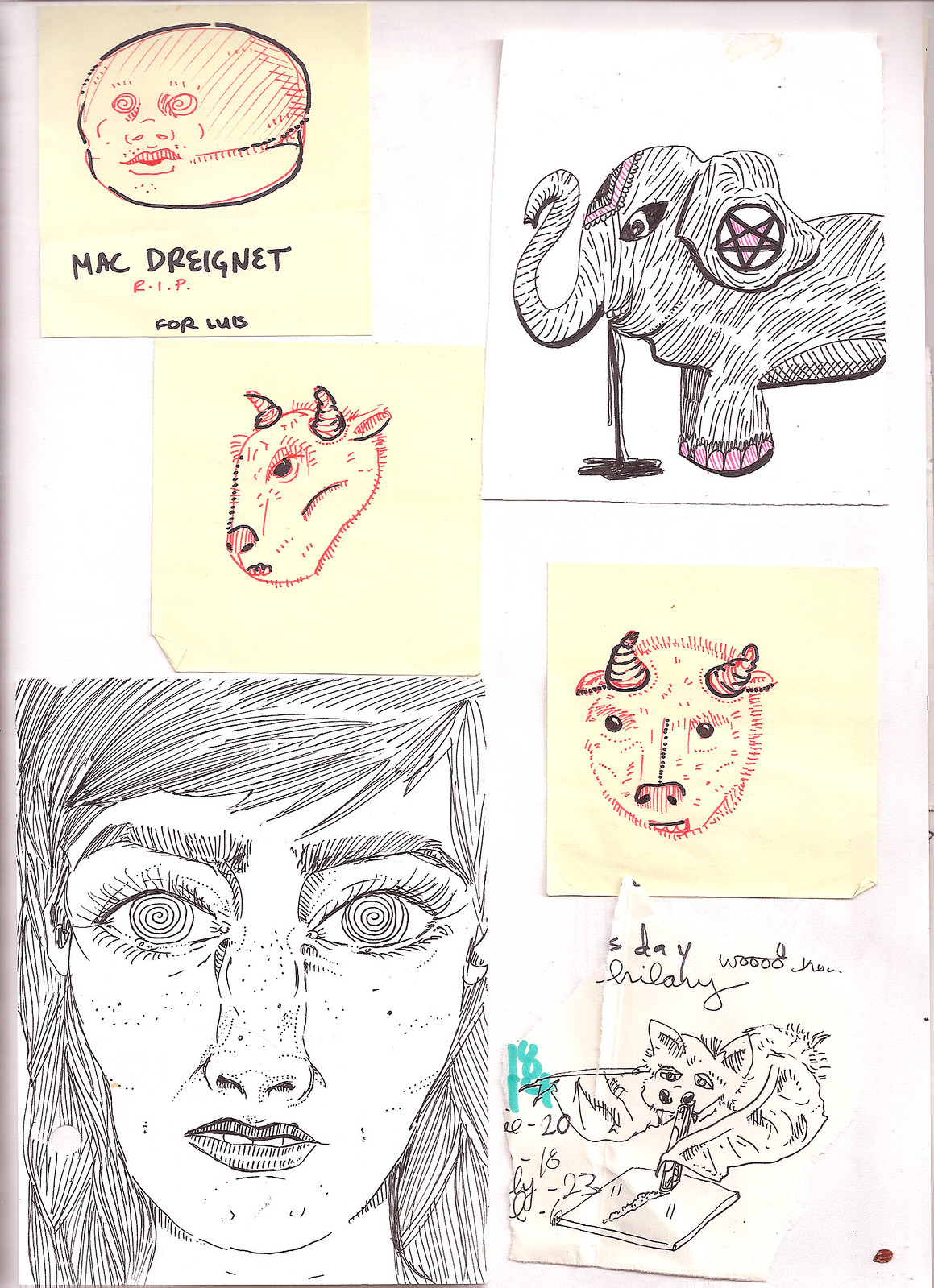This image features a series of six hand-drawn illustrations arranged on a white background. In the upper left quadrant, there is a drawing of a hamburger with a confused face, accompanied by the text "Mac Drainé" or "Mac Dregnet RIP for Lewis". Adjacent to this, in the upper right corner, is an illustration of an elephant with a pentacle on its left ear and pink toenails. The center of the composition contains two horned figures, depicted in black and red line strokes. Moving to the lower left corner, a black pen drawing of a close-up of a woman's face with spiral irises is situated. In the bottom right, there is a drawing of a bat or wolf-like creature with partial text reading "day woo now Friday 2018 by 23". The illustrations feature a mix of colors including black, white, yellow, and red, each on its own square piece of paper. The overall layout and artistic style suggest a curated collection of individual sketches displayed together.